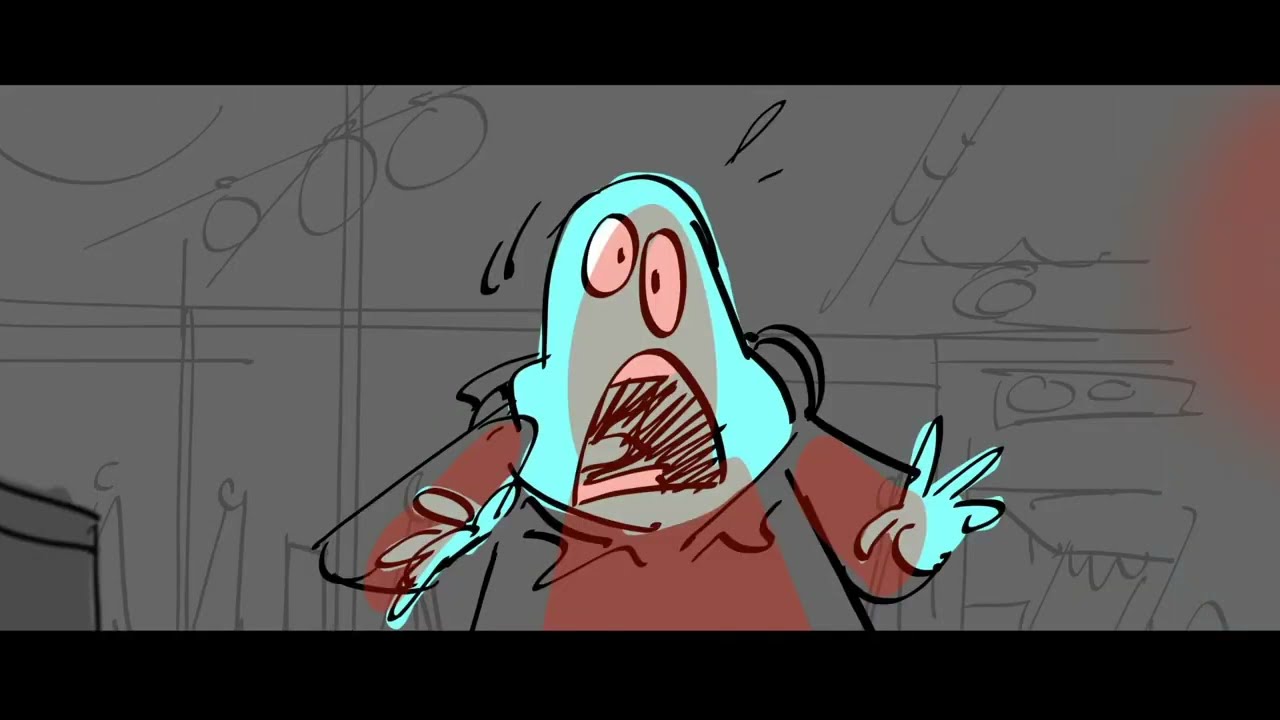A rough storyboard sketch depicts a shocked character with light blue skin and no hair, likely an alien or monster. The character is facing the camera but looking slightly past the viewer, with a shadowy red silhouette cast on his face. His wide-open mouth suggests he's screaming in terror, complemented by his offset eyes, with the left eye positioned higher and the right one drawn longer and lower. He wears a dark robe-like garment and his hands are outstretched defensively, as if warding off a threat. The background is sparsely detailed with gray sketches, showing rough silhouettes of people on the left, resembling cones with circles atop, a light post with two rods and three circles, and other indistinct elements. The character’s distress is further highlighted by an added sweat bubble above his head and the vivid contrast of his blue skin against the otherwise monochromatic scene.